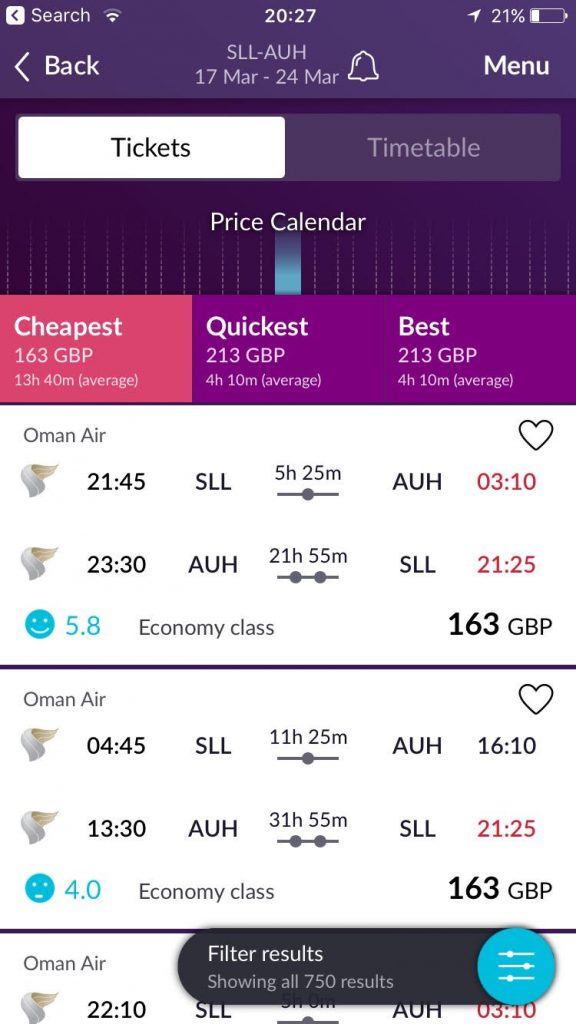Detailed Caption:

The screen displays a ticket reservation interface on a cell phone. The top section has a purple background featuring a white text label "Search" accompanied by a small box with a purple arrow pointing left. Icons for search and volume control appear in white. The current time is shown as "20:27" on the left, while the battery status is indicated on the right as "21%" with an outline colored to match.

Centered in the middle in gray text, the section displays "SLL-AUH, 17 March to 24 March" alongside a bell icon. A back arrow icon in white is located on the left, and "Menu" is on the right.

Below, the interface is divided into two distinct banners. The first banner, predominantly white with a purple section on the right, reads "Tickets" in black and "Timetable" in gray. The next banner lists "Price Calendar" in white text with a blue vertical line. It categorizes options as "Cheapest," "Quickest," and "Best." "Cheapest" is highlighted in a pink box reading "163 GBP, 13 hours 40 minutes average," "Quickest" and "Best" both list "213 GBP, 4 hours 10 minutes average."

A fine black line separates the above elements from the listings below. The first listing on a white background details a flight from Oman Air, scheduled at "21:45 SLL, 5 hours 25 minutes" to "AUH." It marks "03:10" in red and features a black outline heart above. Another line reads "23:30 AUH, 21 hours 55 minutes" to "SLL" with "21:25" in red. Information describes "Economy Class, 5.8" with a blue smiley face and a fare of "163 GBP."

Following another thick black line, the second entry describes an Oman Air flight departing "04:45 SLL, 11 hours 25 minutes" to "AUH" arriving at "16:10," again marked with a heart icon. Another leg appears as "13:30 AUH, 31 hours 55 minutes" to "SLL" with "21:25" in red. It is described as "Economy Class, 4.0" with a blue frowning face and "163 GBP."

The final entry, separated by a thick black line, notes an Oman Air flight leaving at "22:10 SLL" destined for "AUH" marked at "03:10" in red. A black popup banner overlays part of the text stating "Filter results" in white, indicating "Showing all of 750 results" with a clickable blue circle featuring three horizontal lines for additional options.